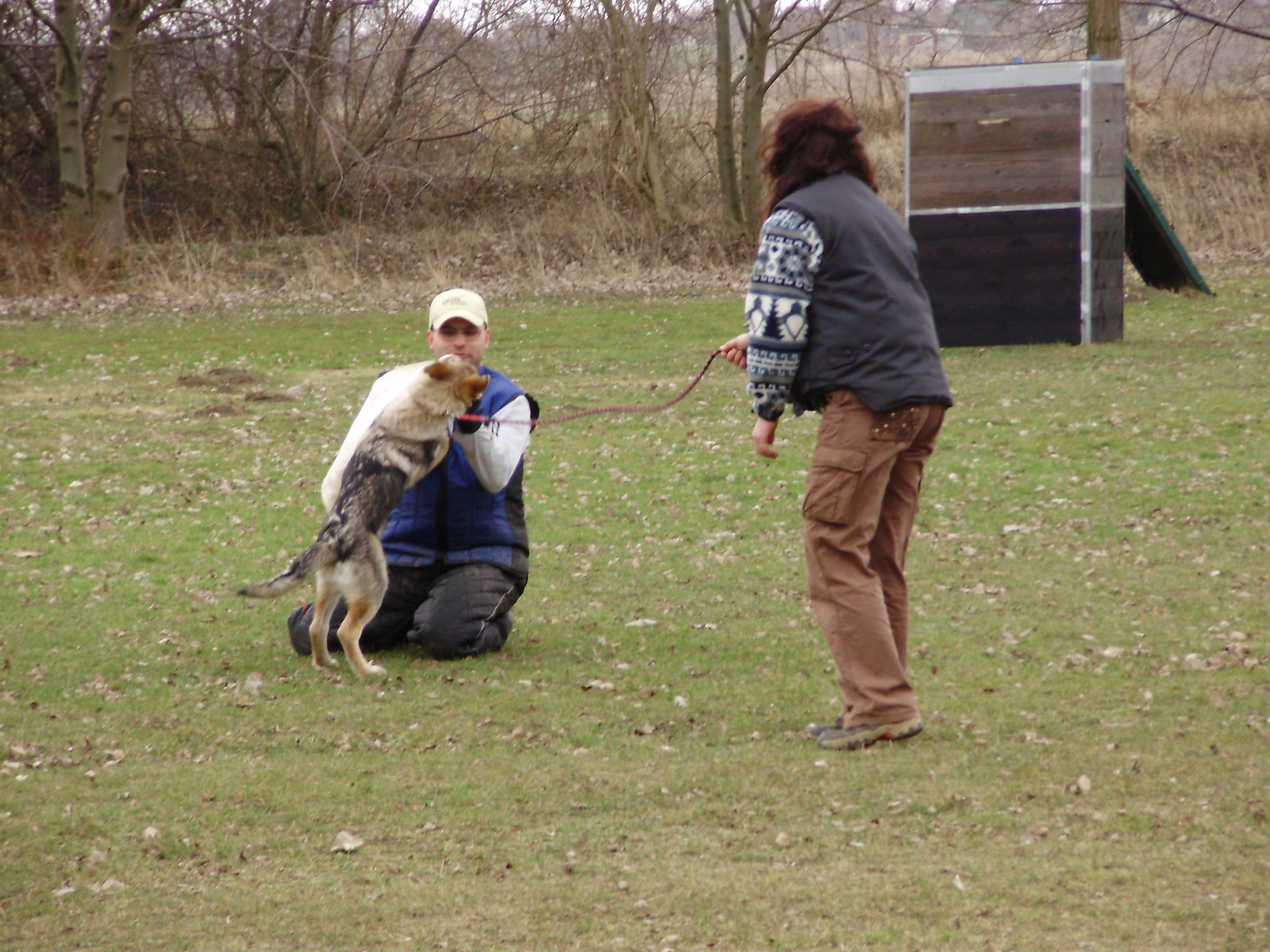In an open field sprinkled with scattered, fallen leaves, likely indicating it's fall, two white individuals are interacting with a dog in front of a line of leafless trees. The woman, dressed in a winter sweater overlaid with a gray vest, and brown pants, is holding a leash attached to the dog. She stands to the right, observing the scene. The man, wearing a protective white long-sleeve shirt, a blue vest, a white baseball cap, and kneeling on the grass, is engaging with the dog. The dog, standing on its hind legs with its front paws pressed against the man, appears to be in training. A vertical plank of wood protrudes in the background, adding a rustic element to the otherwise natural setting.